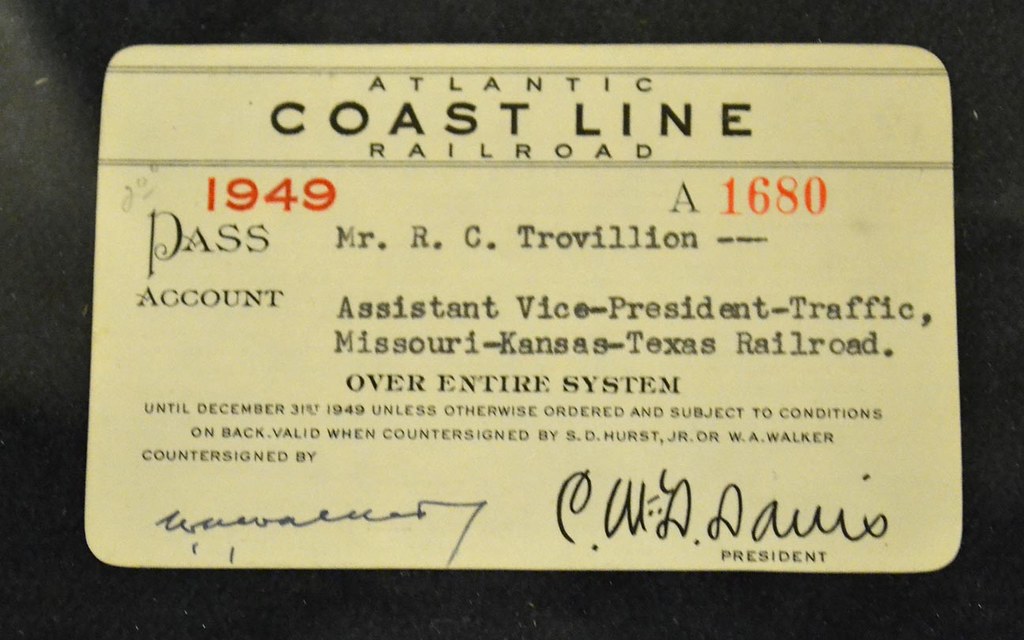The image showcases a vintage, light beige ID card with rounded corners set against a dark gray background. At the top center of the card, it reads "Atlantic Coastline Railroad" in bold lettering. Below this, aligned to the left, are the numbers "1949" in red, followed by a black "A" and "1680" in red numerals. Underneath these details, the word "Pass" is followed by the typed name "Mr. R. C. Trevelyan, Assistant Vice President of Traffic, Missouri-Kansas-Texas Railroad." The card states "Over entire system until December 31st, 1949 unless otherwise ordered and subject to conditions on back." It specifies the pass is "valid when countersigned by S. D. Hearst, Jr. or W. A. Walker." At the bottom, there are two handwritten signatures; the one on the left is illegible and possibly reads "Walker," while the right one is clearer, appearing to be "C. W. D. Davis," beneath which is the title "President."